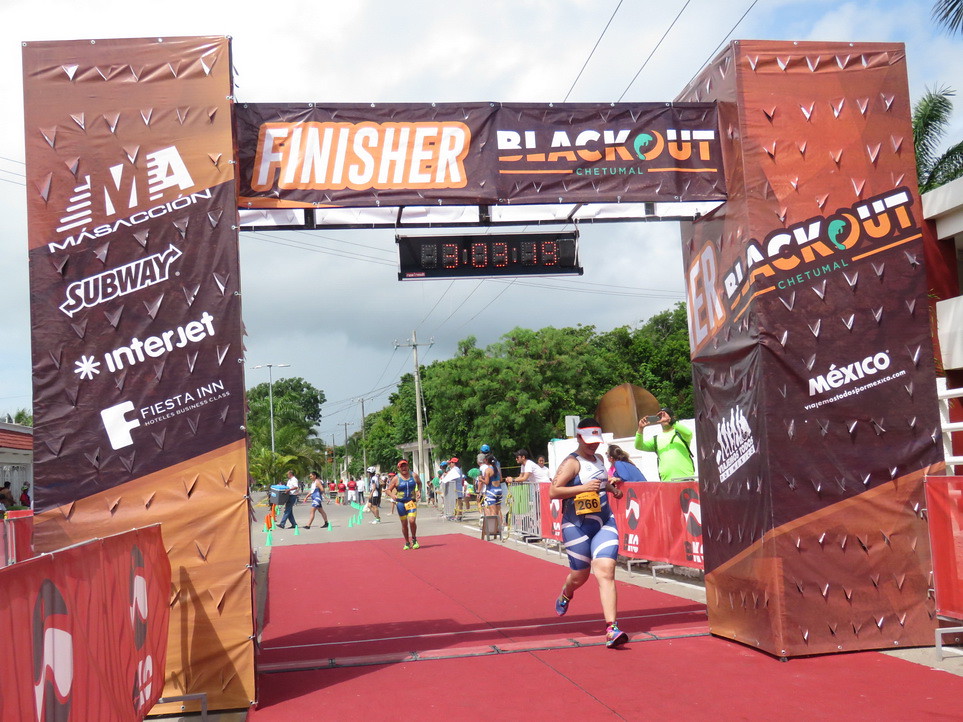The photograph captures the climactic finish of a foot race. Dominating the scene is a portable finish line, held aloft by two upright portions with a brown and dark red color scheme, embellished with sponsor logos such as Subway, Interjet, and various other Mexican brands. The banner overhead reads "FINISHER" in bold white letters with a gold drop shadow, followed by the words "Blackout" and "Chet Yumal." Suspended from the banner is a digital clock displaying a time of three hours, three minutes, and nineteen seconds. A red carpet unfurls across the road, guiding the racers towards their goal.

In the foreground, a runner wearing a blue and white striped outfit, marked with the number 266, crosses the finish line. Behind them, more competitors are visible, one notable runner in the background sporting a gold placard and purple shorts. The race is framed by vibrant green trees and a partly cloudy sky, adding a touch of natural beauty to the bustling scene. Spectators stand behind guardrails, cheering the athletes on as they complete their journey in this vivid, action-packed moment.